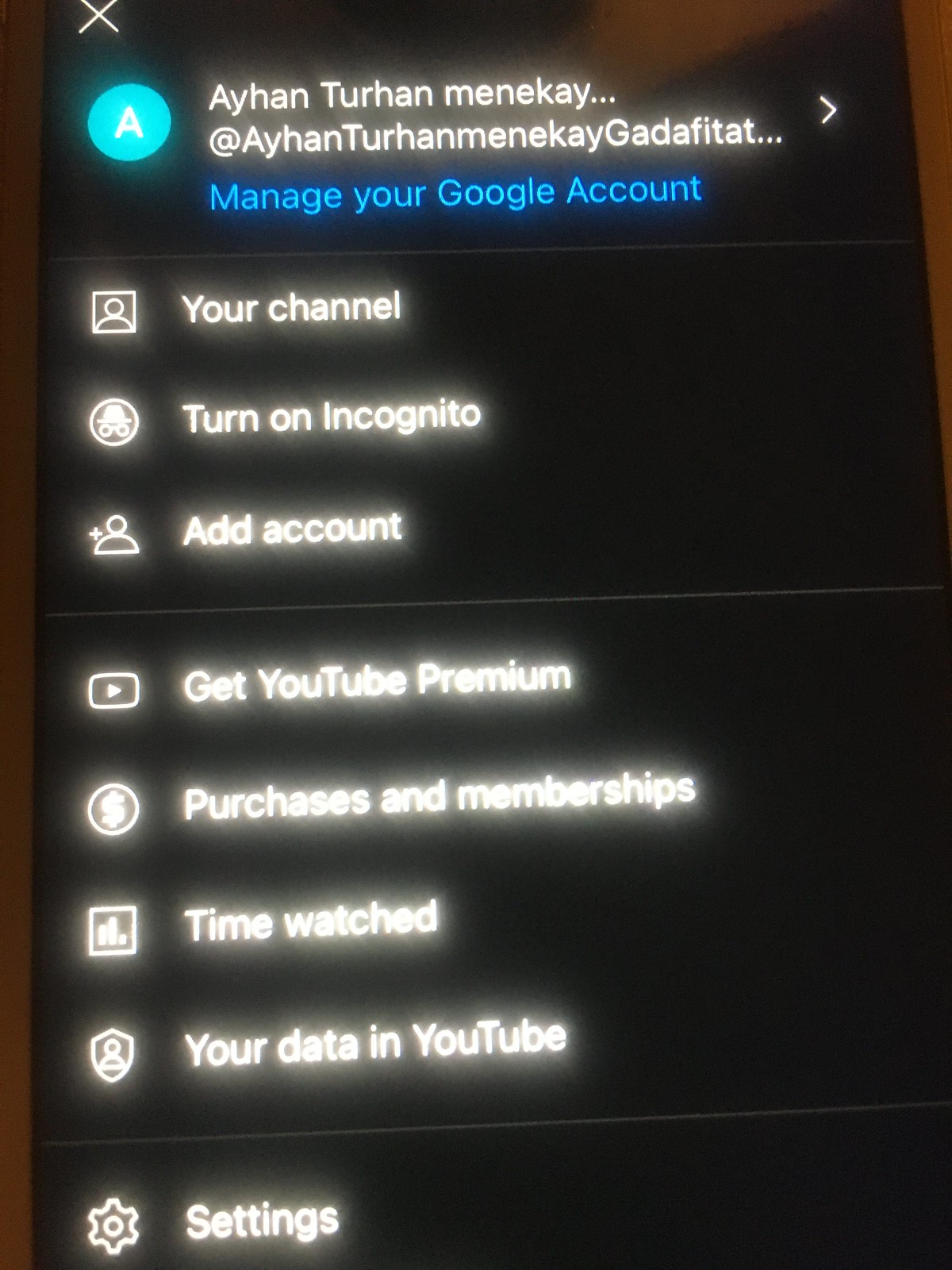This image depicts the settings menu of a Google Account, showcasing various user management options on a dark-themed interface. The background is black, indicating the night theme is active. 

At the top left, there's a blue circle with a white 'A' in it, representing the user's profile icon. Next to it is the user's name, "Ahan Turnam," followed by an '@' symbol and a lengthy username. Just below the name, highlighted in blue, is an option labeled "Manage Your Google Account," with an arrow pointing to the right.

The menu is organized into several sections:

1. **Profile and Channel Management**:
   - **Your Channel**: Represented by an icon featuring a portrait frame and a stick figure.
   - **Turn on Incognito**: Marked by an icon of a hat and glasses within a circle.
   - **Add Account**: Indicated by a round head with a '+' sign.

2. **YouTube Specific Options**:
   - **Get YouTube Premium**: Illustrated with a play button icon.
   - **Purchases and Memberships**: Depicted by a circle with a dollar sign.
   - **Time Watched**: Symbolized by three bar graphs within a square.
   - **Your Data in YouTube**: Looking similar to a badge.

3. **General Settings**:
   - **Settings**: Represented by a gear cog icon, situated in a separate section at the bottom of the menu.

This detailed layout provides users with a comprehensive overview of the management and settings options available for both their Google and YouTube accounts.